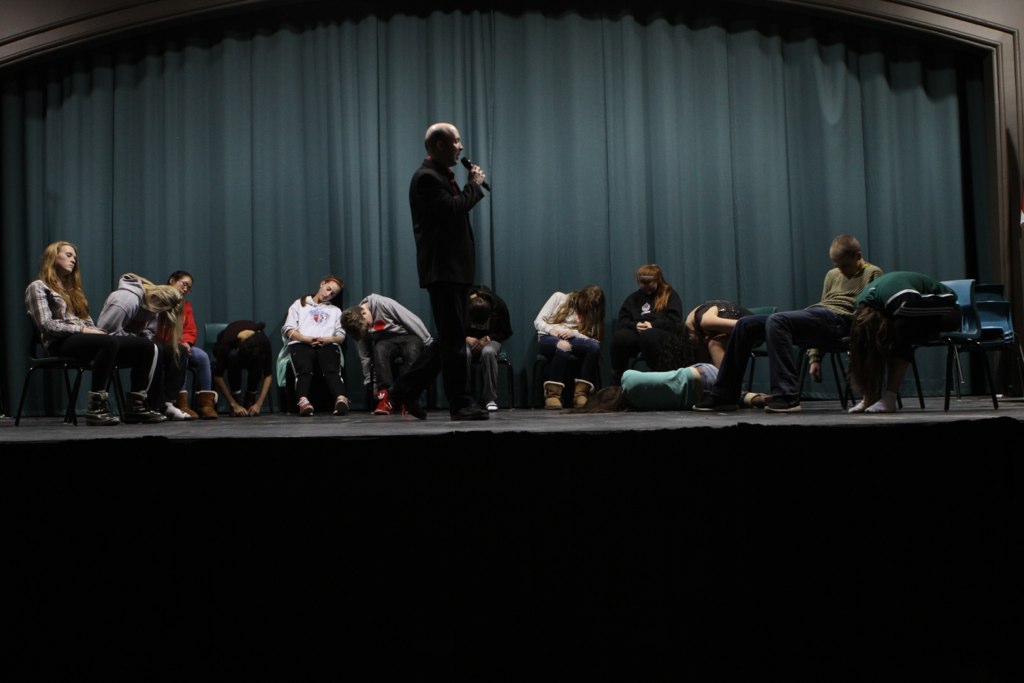In this indoor photograph, the scene captures an audience's view of a dimly lit stage with a large, dark bluish curtain as the backdrop. Center stage stands an older, partially bald man dressed in a black suit that extends to his wrists and holds a microphone in his right hand. He faces to his left. Surrounding him in a circle are at least twelve students, appearing to be either teenagers or of college age. Most of them are slumped over in their chairs, giving the impression that they are either asleep or on the verge of falling asleep. One student, distinguishable by her teal shirt and blue jeans, has even collapsed onto the floor, with long hair obscuring her face. Another student on the far left is less slouched compared to the others but still appears to be asleep. The stage's bottom area remains shrouded in darkness, making it difficult to discern additional details. The overall scene conveys a sense of lethargy and disinterest among the students as they sit around the speaker.